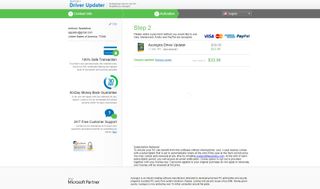This image is a detailed screenshot from a website page instructing how to update a driver. At the top of the page, a gray navigation bar spans horizontally, featuring the text "Driver Updater" in blue on the left side. Below this is a green progress bar, indicating the completion of two steps (Step 1 and Step 2) with Step 3 still pending, highlighted in black.

The webpage is divided into two vertical columns. The left column showcases various icons in blue and green hues. At the top is an icon resembling a card, featuring a green circle at the lower right corner with a number inside. Below this icon, there is another circular icon, divided into thick blue and green semi-circular outlines, and a question mark icon accompanied by a small box beneath it.

On the right column, the section for Step 2 is prominently displayed in bold green font. Beneath this heading, a descriptive text is printed in black. Below the description, payment method icons are lined up: Visa in blue, MasterCard in red and yellow with interlocking circles, American Express in blue, and PayPal italicized. An item has been added to the cart, with its pricing clearly displayed. At the bottom of the page, a gray bar spans horizontally, containing a disclaimer.